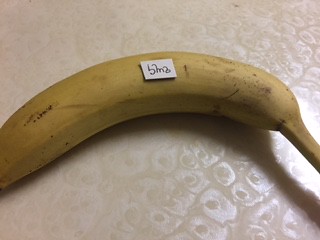The image is a close-up, almost bird's-eye view photograph of a banana resting horizontally on a white, textured surface that resembles a tablecloth or possibly a countertop with a circular pattern. The banana stretches from the left to the right side of the image, curving slightly downwards. Only about 90-95% of the banana is visible, with the tips cut off by the edges of the photo. The banana is partially ripened, showing a deepening yellow color interspersed with brown and black spots. At the center of the banana, there is a small rectangular white label with indistinct black lettering that resembles "5M0," "5M2," or "BLMA." The surface beneath the banana has a slight glare, giving it a bit of a shine, and the banana casts a shadow predominantly on the right side.